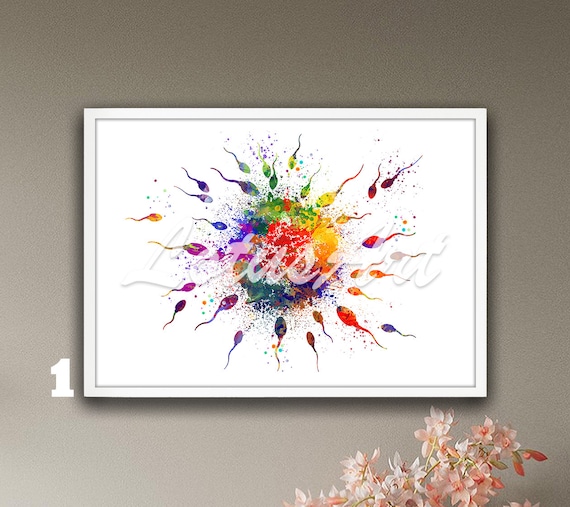The image captures a striking piece of artwork hanging on a light gray, textured wall, likely in an art gallery. The artwork, set within a white-bordered frame, showcases a vivid scene of multicolored sperm cells, covering the full spectrum of the rainbow, flying radially towards a multi-hued egg in the center, all against a pure white background. There's ghostly, almost transparent text superimposed on the image, centered around the colorful egg, and though it's difficult to read, one might discern a "U" and an "S." Below the artwork, near the bottom right edge of the frame, a pinkish plant extends upward, adding an organic touch to the composition. Additionally, the number "one" is visible on the wall to the left of the frame, enhancing the gallery-like setting of this compelling piece.